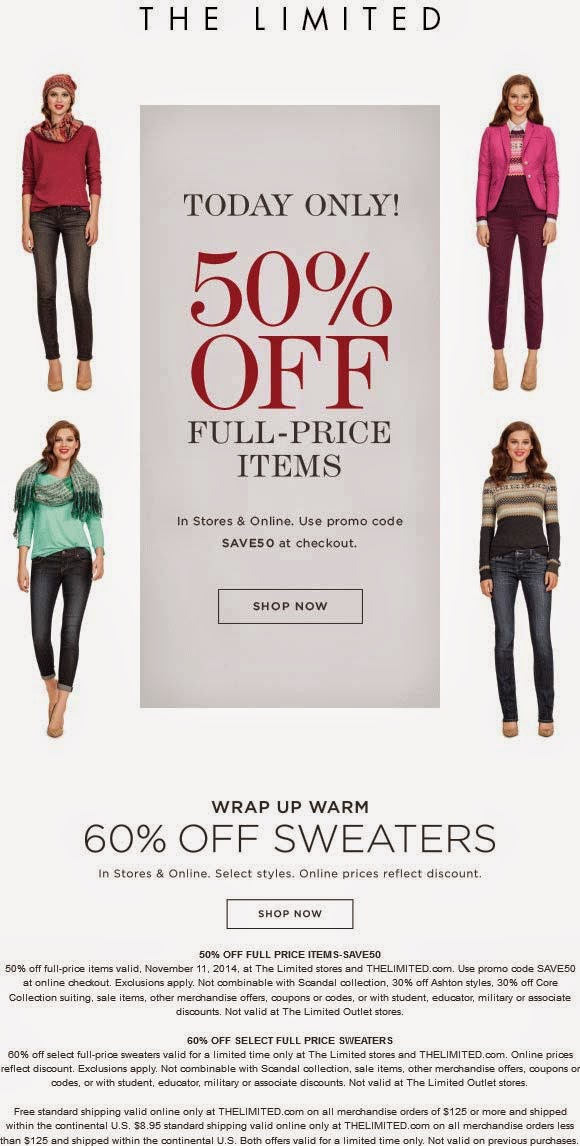In this advertisement from a clothing website, we have a predominantly whitish light gray background. The ad features images of the same woman styled in four different outfits. On the left side of the ad, she appears once at the top and once at the bottom. Similarly, on the right side, she is featured once at the top and once at the bottom.

At the very top of the ad, the word "Limited" is written in black. In the center of the image, there is a vertically aligned gray rectangle. The text inside the rectangle reads "Today Only 50% Off" in red, followed by "Full price items in stores and online. Use promo code SAVE50 at checkout." Beneath this, there is a "Shop Now" button.

Below the central gray rectangle, another promotion is presented: "Wrap Up Warm" with "60% off sweaters in stores and online, select styles." It also notes, "Online prices reflect this discount." Another "Shop Now" button is positioned below this promotion. At the bottom of the ad, the terms and conditions of the discounts are written in fine print.